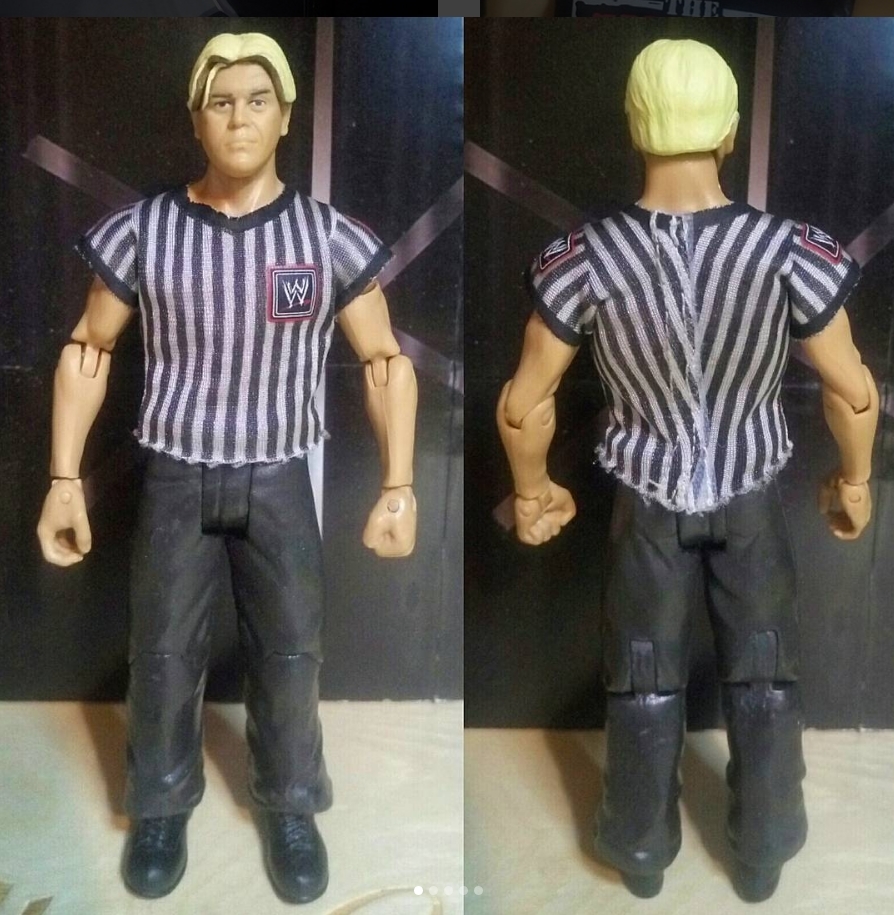The image is a composite of two photographs, presenting the front and back views of an action figure. On the left side, the action figure faces forward, revealing its attire: a black and white vertical striped shirt reminiscent of a referee's uniform, adorned with a WrestleMania logo on the left breast. The figure also wears black pants and black shoes. The arms are articulated with distinct sections for the bicep, forearm, and wrist, allowing for movement. The figure is characterized by its blonde hair, parted in the middle. On the right side of the collage, the back view of the action figure is displayed, providing a complete perspective. The setting features a white floor and a black wall with stripes in the background, adding to the visual distinction of the figure.